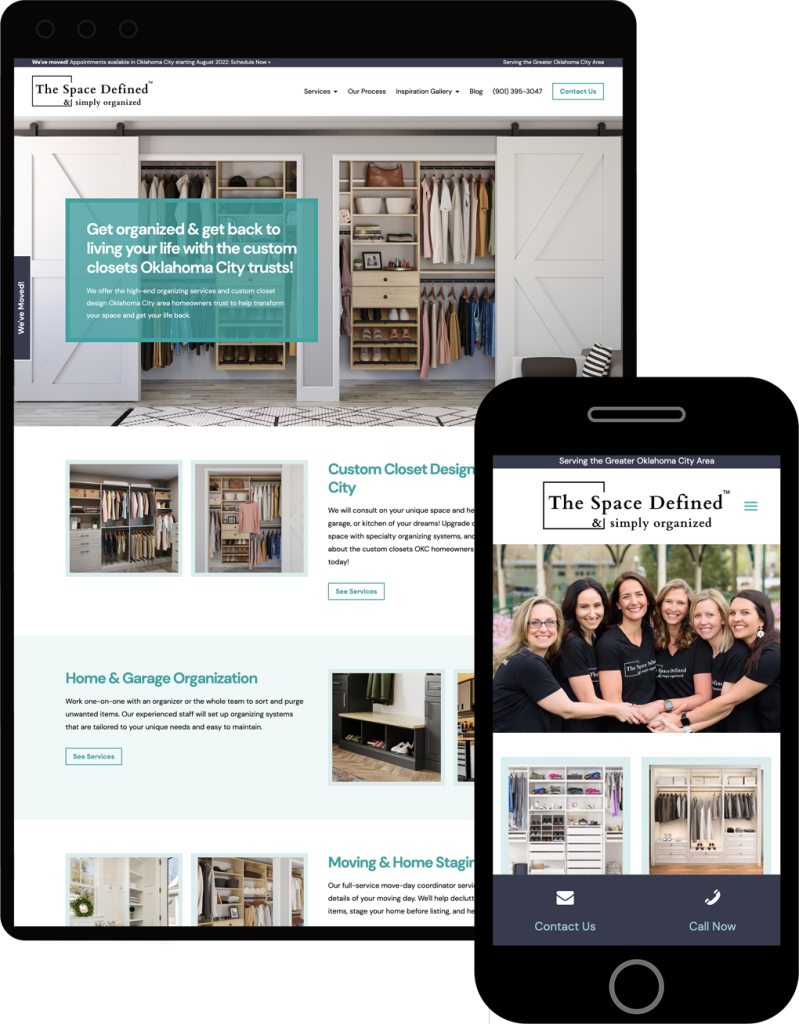The image features two black smartphones displaying promotional content for a custom closet design company in Oklahoma City. The first phone at the top shows:

1. A small blue line with tiny white text.
2. A prominent white box with the text "The Space Defined" and a marked square.
3. Several small topics listed underneath, including a "Compare Us" button.
4. A visually appealing image of a closet with a large green box in the center containing the text: "Get organized and get back to living your life with the custom closets Oklahoma City trusts."
5. A small gray tag with white print on the left side of the image.
6. Below this, a large white box featuring two additional images and the phrase "Custom Closet Design".
7. A small blue box mentioning "Home & Garage Organization" with related images on the right side.
8. Several smaller images at the bottom relevant to home organization.

The second phone displays:

1. A gray strip across the top stating "Serving Greater Oklahoma City."
2. A large white box titled "The Space Defined, Simply Organized" with a block around it.
3. An image of six women.
4. Another large white box featuring two closet images.
5. A gray box with "Contact Us" and "Call Now" options.
6. The phone encircled in a distinct black ring in the middle.

Together, these elements showcase the services and features of the custom closet company, emphasizing organization and design.